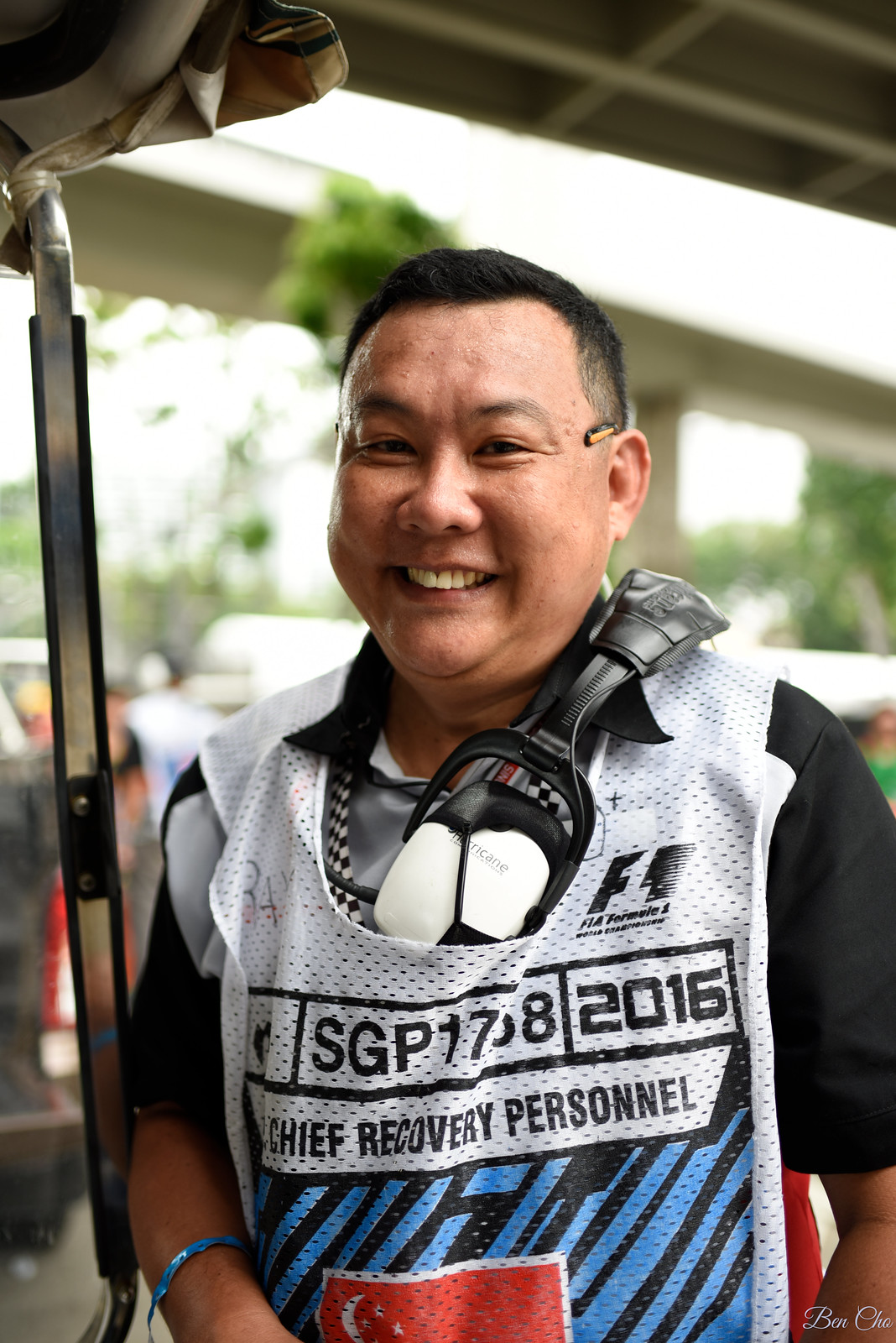The image depicts an Asian man in his 40s standing outdoors during the day against a blurred background of trees and possibly some roadway elements. He has a wide face, high forehead, and short black hair, wearing no glasses but holding something behind his ear. A pair of headphones hang over his left shoulder, and he sports a blue bracelet on his right hand. The man is smiling warmly at the camera, dressed in a black t-shirt under a black-and-white plaid shirt, and further covered by a distinctive vest. The vest is predominantly black and white with blue stripes, emblazoned with the text "SGP-17-2016 Chief Recovery Personnel" and "FTA" on the top right corner. An emblem resembling a red flag with a yellow crescent and stars, suggesting affiliation with China, is also visible on the vest. The overall scene is set against a backdrop hinting at trees and a gray sky.